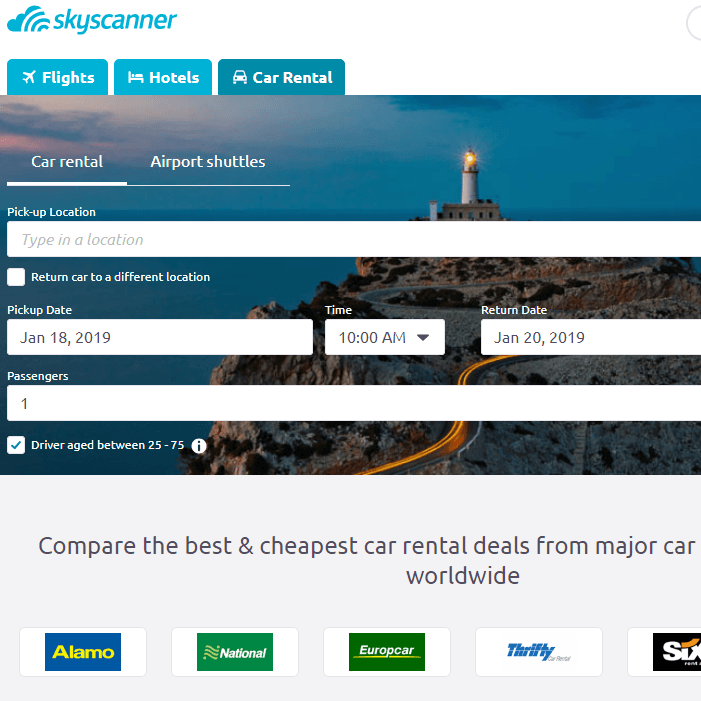In the image, the top left showcases a cloud with pronounced white lines cutting through it, set against a sky scanner interface featuring a prominent blue button labeled "Flights." Adjacent to this button, options for "Hotels" and "Car Rental" are visible, with the white text clearly displaying "Car Rental." There are additional options for "Airport Shuttles" as well. 

A lighthouse stands tall beneath a dark sky, accessible via a windy road that leads up to it. Below this scenic depiction, there is a section labeled "Pick Up Location" with fields to "Type in Location," "Type in a Location as We Told Them," and other pertinent information in gray text.

A large white square contains essential booking details: "Return Car to a Different Location," "Pick Up Date: January 18th, 2019, Time: 10 AM," "Return Date: January 20th, 2019," "Passengers: One," and "Driver Age: Between 25 to 75."

The image also promotes checking and comparing the best and most affordable car rental deals from major companies worldwide. A blue label indicates "Alamo," a green square signifies "National," followed by "Europcar" with the number 30, and another unspecified black square likely representing an additional rental option.